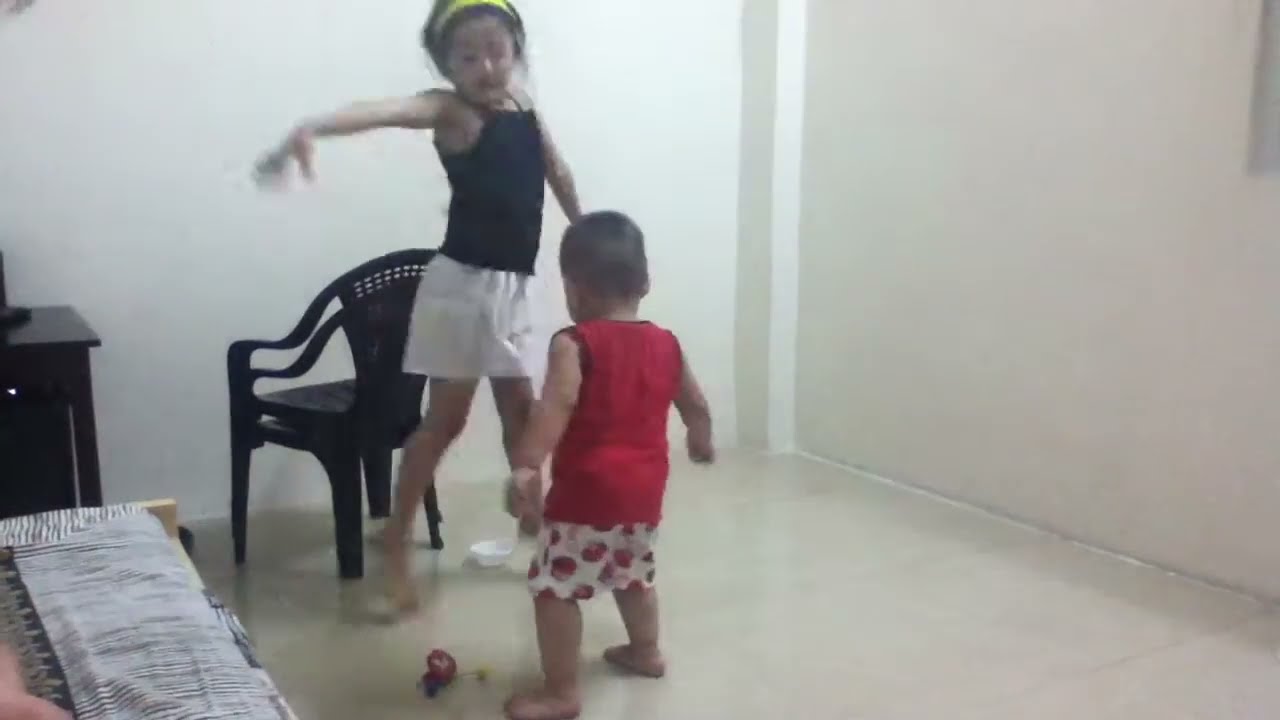In a white room with gleaming, off-white floors, two young children, who appear to be Asian, draw attention with their vibrant energy. The girl, around seven or eight years old, dressed in a black tank top, white shorts, and a neon yellow headband, is captured mid-air with her arms outstretched, as if dancing or jumping. She has black hair and is positioned towards the left side of the frame. Behind her stands a stack of two black plastic lawn chairs. To the very left, a wooden cabinet is visible. In the foreground, a younger boy, approximately three to four years old, stands firmly on the ground, barefoot and focused on the girl's movements. He wears a red tank top and white shorts with red patterns resembling cherries. A toy lies on the floor in front of him. The serene white walls and simple decor emphasize the children's playful interaction, making them the focal point of the scene.